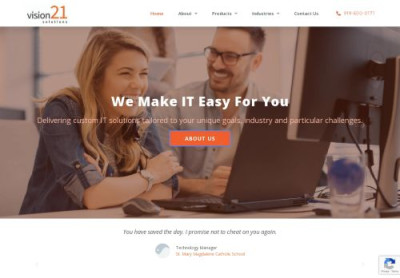"Homepage of Vision 21 website featuring a clean, white background with black menu options at the top. The prominent focal point is a vibrant photo of two individuals sitting together at a computer, both smiling and appearing to collaborate on a computer-related task. The text overlay in the main section reads, 'We make IT easy for you. Delivering custom IT solutions tailored to your unique goals, industry, and particular challenges.' An eye-catching orange 'About Us' button is positioned below this text. A variety of additional information and options are presented at the bottom of the page, accompanied by the circular Kapska logo in the bottom right corner, designed with multiple shades of blue and gray. A prominently displayed telephone number in orange adds a touch of accessibility to the site."